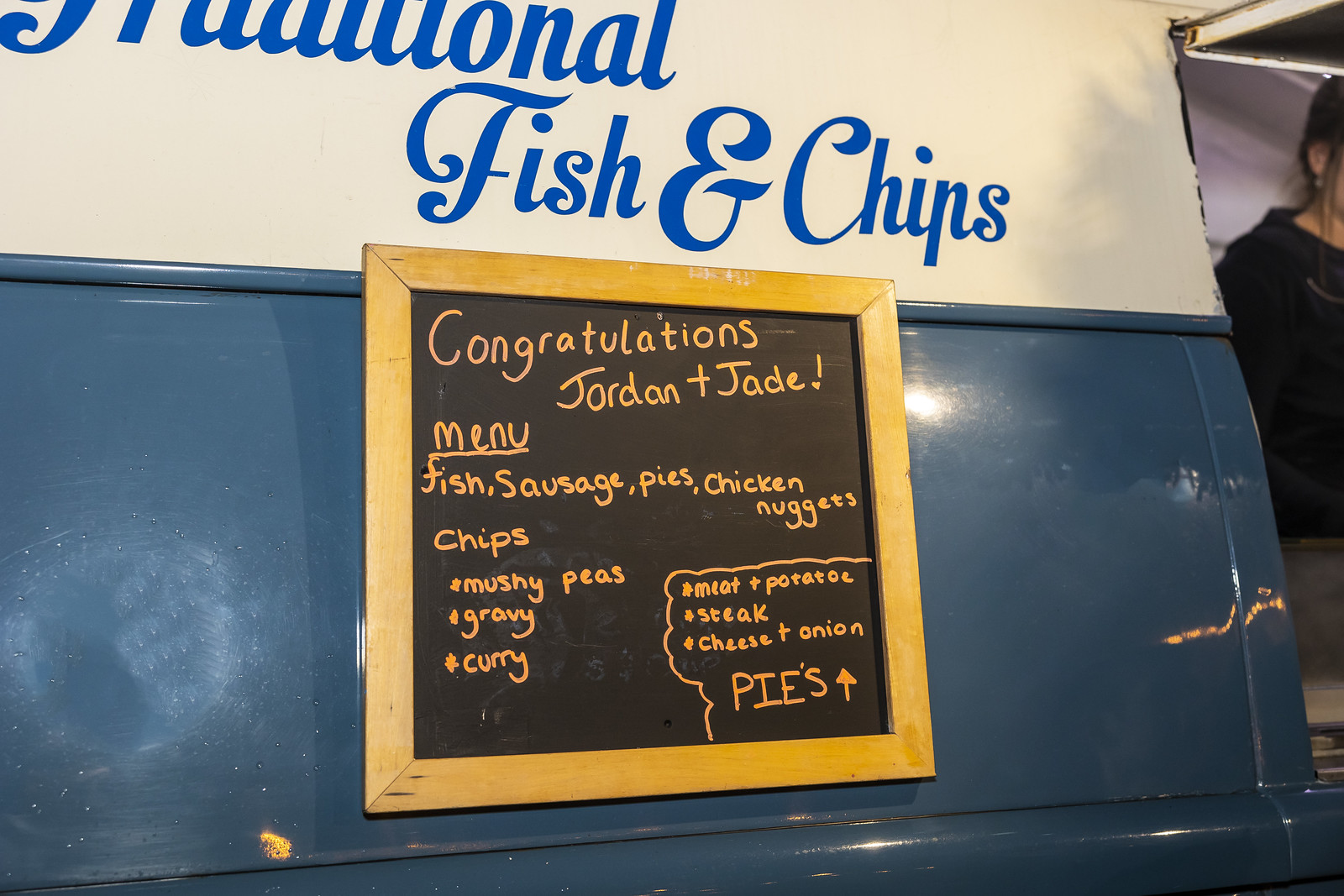The image features an outdoor scene of a food truck. On the far right, a person with dark clothing and dark hair stands, their face not visible. The food truck itself has a white upper section with blue cursive writing that partially reads "Traditional Fish and Chips." Below this, the lower half of the truck is painted blue and features a chalkboard with a wooden frame. The chalkboard has a black background with gold-colored writing. It reads: "Congratulations, Jordan and Jade," followed by a menu listing items such as fish, sausage, pies, chicken nuggets, chips, mushy peas, gravy, and curry. In the bottom right corner of the chalkboard, additional items are listed with an arrow pointing up: meat and potato, steak, and cheese and onion pies.